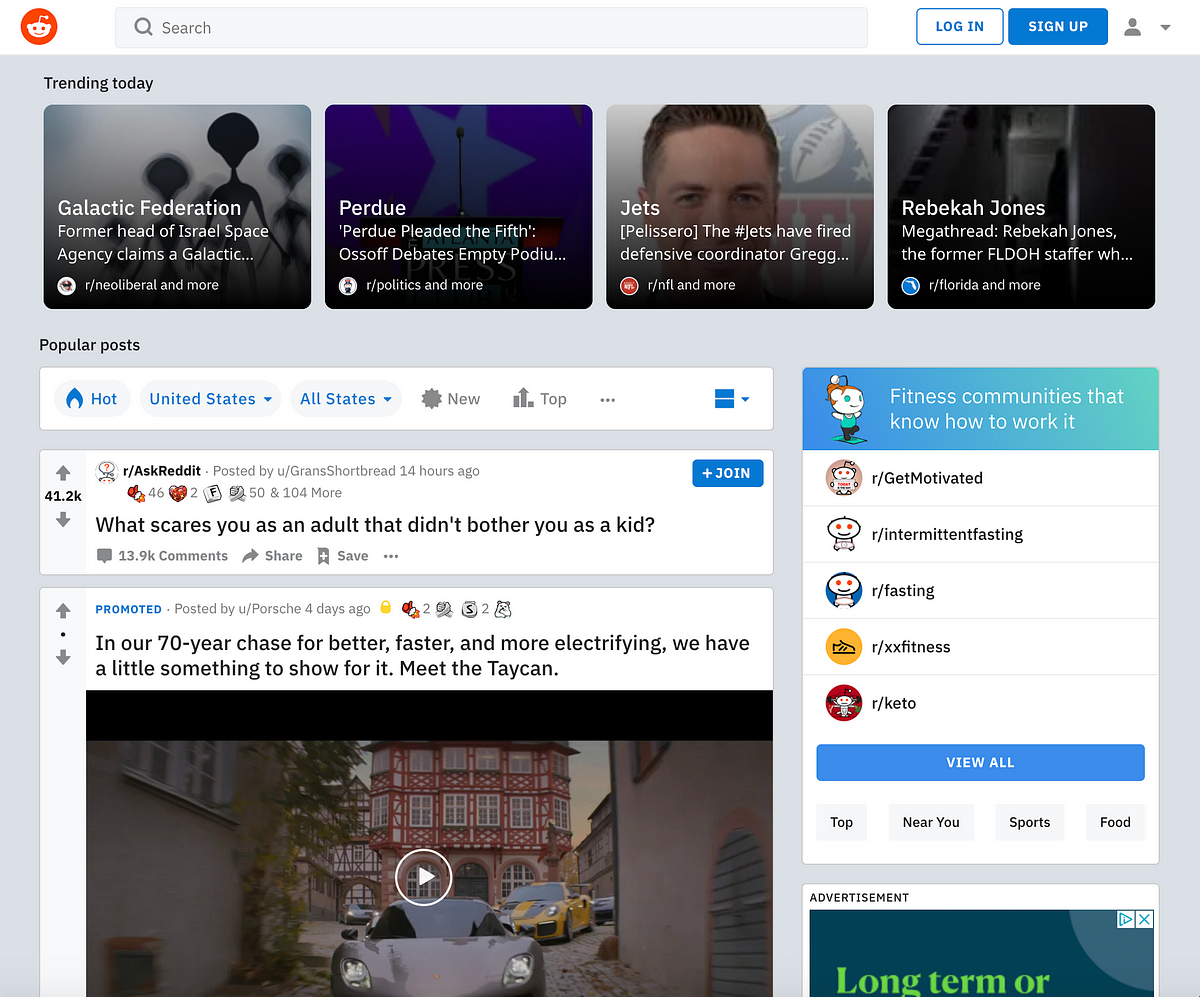**Screenshot Description:**

The screenshot captures a web page of the popular social media platform Reddit.

---

1. **Top Section:**

At the top left corner, the iconic Reddit logo is visible – an orange-red circle featuring a white alien face. Directly next to the logo is a magnifying glass icon, followed by a search bar with the placeholder text "search." To the right of the search bar is a white box with a blue outline containing the word "login" in blue letters. Adjacent to this is a blue box with "sign up" in white letters. Additionally, there's a small person icon accompanied by a dropdown arrow.

2. **Main Content:**

- Beneath this top section is a gray box containing various content cards.
  
  - **Trending Today:** 
    - **Top Left Content Card:**
      - Thumbnail and text for "Galactic Federation" with the headline: "Former head of Israel Space Agency claims a galactic…" indicating it's from the subreddit r/neoliberal and possibly others.
    - **Top Right Content Card:**
      - Thumbnail for "Purdue," with the description: "Purdue pleaded the fifth, Ossoff debates empty podium," linked to r/politics and more.
    - **Bottom Left Content Card:**
      - Thumbnail of a person's face with the NFL shield, headline: "Jets [Pellicero] The #Jets have fired defensive coordinator Greg…" linked to r/NFL and more.
    - **Bottom Right Content Card:**
      - Thumbnail for Rebecca Jones, headline: "Rebecca Jones megathread, the former FLDOH staffer…" linked to r/Florida and more.

3. **Side Navigation:**

- On the left-hand side is a section headlined "Popular Posts." Below this is a white box with:
  - A blue flame icon labeled "hot" and dropdowns set to "United States" and "all states."
  - Grayed out icons for "new" and "top" posts, and an option represented by three horizontal dots.

4. **Highlighted Post:**

- Below the side navigation:
  - **Post by r/AskReddit:**
    - Voting arrows on the left with a count of 41.2K in between.
    - Title: "What scares you as an adult that didn’t bother you as a kid?"
    - Posted by user grands shortbread 14 hours ago.
    - On the right, a blue button labeled "join" and several interaction icons.
  - Comment count: 13.9K
  - Share option, save option, and an additional menu represented by three horizontal dots.

- **Promoted Content:**
  - Indicated by blue text "promoted," attributed to user Porsche (the car company).
  - Title: "In our 70-year chase for better, faster, and more electrifying, we have a little something to show for it; meet the Taycan," with an embedded video.

5. **Additional Content:**

- To the right are links to "Communities that know how to work it," including subreddits like r/GetMotivated, r/Intermittent Fasting, r/Fasting, r/XXFitness, and r/Keto, with a "view all" button.
- Categories for browsing: Top, Near you, Sports, and Food.

6. **Advertisement:**

- At the bottom right corner, there's a partially visible advertisement box indicating an advertisement with a cut-off phrase "long-term or…" in green text.

---

This detailed descriptive caption encapsulates the structure and content within the screenshot, providing an intricate breakdown for a comprehensive understanding.